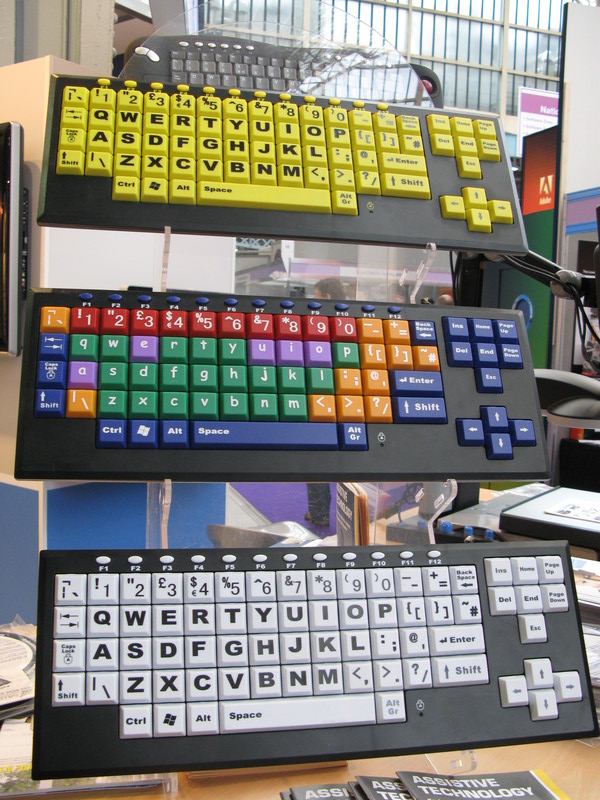A detailed photograph taken indoors features three distinct keyboards mounted vertically on a clear plastic display case. The display is set against the backdrop of a large office building, with various computer equipment and accessories visible in the background. 

The bottom keyboard boasts a gray base with white keys, featuring large, bold black text for letters, numbers, and symbols. The middle keyboard, in contrast, has a black base and colorful keys. It displays a striking array of colors: red numbers, green consonants, purple vowels, and dark blue function keys like Enter, Shift, and Space. Orange and purple special function keys add to its vibrant palette. 

The top keyboard is characterized by a dark gray base and bright yellow keys, adorned with large, bold black text. Unlike the others, it features the alphabet and basic function keys prominently, excluding the number nine key. The trio of keyboards is prominently displayed, with the bottom edge of the display area showing booklets titled "Assistive Technology."